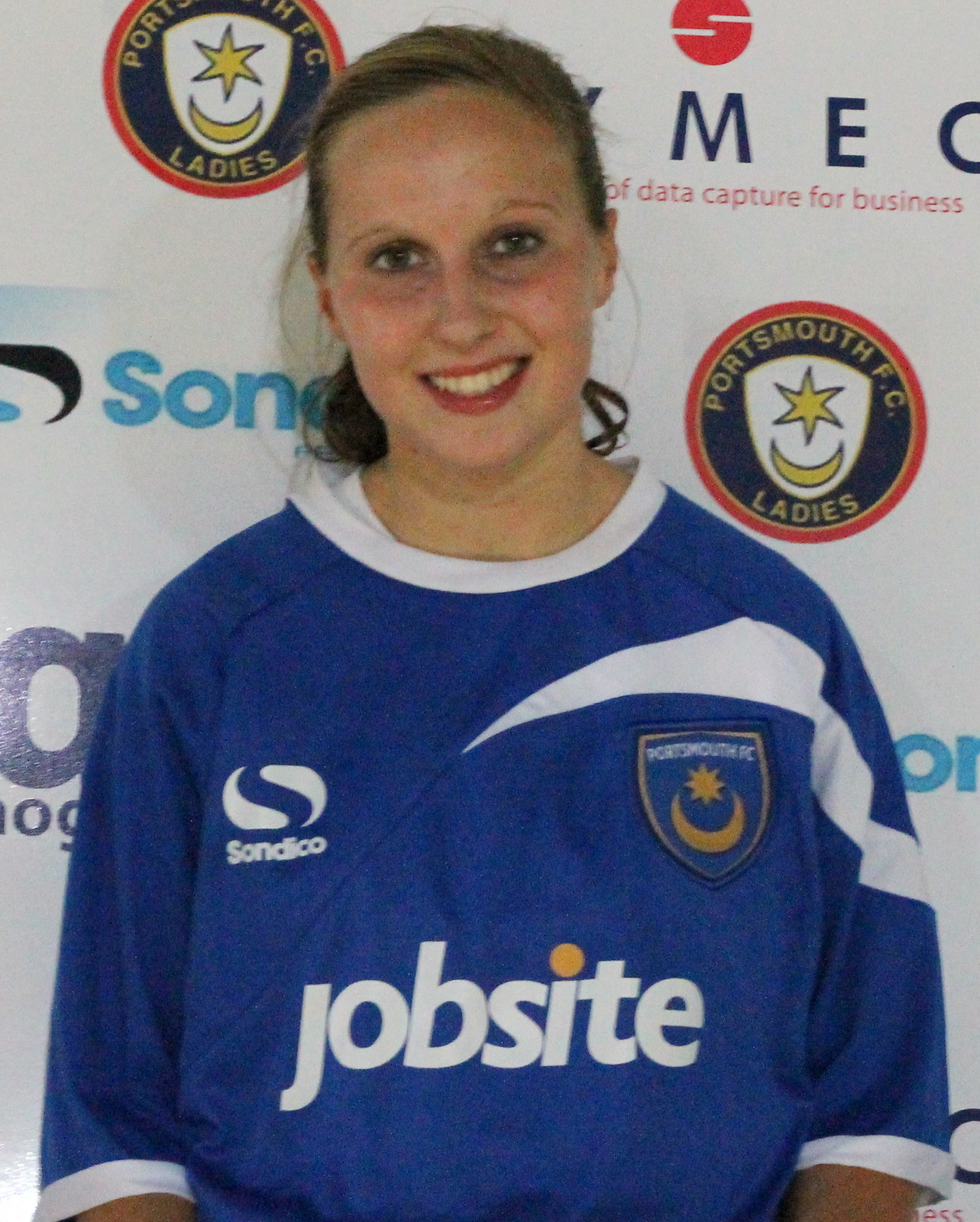In the image, a young woman of Caucasian descent with blonde hair tied back in a messy ponytail is positioned centrally and facing directly at the camera. She is smiling, showcasing red lipstick and the upper row of her teeth. She appears to be in her late teens or early twenties. She is wearing a blue short-sleeved sports jersey that reaches her elbows, featuring a white collar and cuffs. The jersey prominently displays the word "Jobsite" in white text across the front, with a yellow dot above the "i." 

On the left side of her chest, there's a blue shield outlined in gold with "Portsmouth FC" written in white, and below it, a yellow sun with a half moon underneath. The right side of her chest bears the word “Sandico” in white. The background consists of a covered wall filled with logos and text primarily related to Portsmouth FC and its sponsors. Notable visible text includes "Portsmouth FC Ladies" and "data capture for business." The colors in the image are vibrant, including hues of blue, white, yellow, orange, red, and various shades of blue. The setting appears to be indoors, possibly at an award ceremony or a similar event for soccer players.